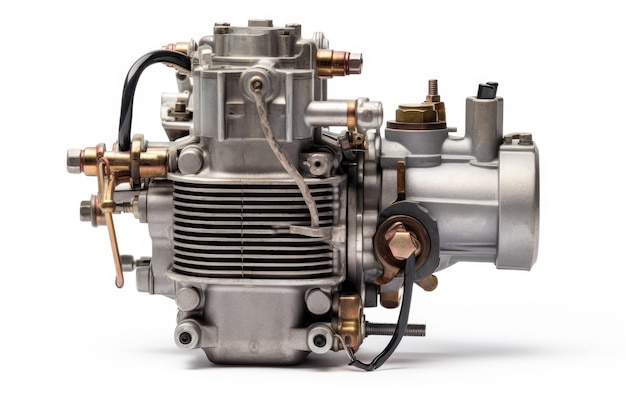The image depicts a side view of an engine set against a white background, with light coming from the left side, casting a slight shadow underneath. The engine is predominantly silver, with various components including black and brass parts. An intricate network of bolts, nuts, and copper fittings are visible throughout the machinery. A prominent feature on the right-hand side is a large, shiny bronze cylinder pointing horizontally, connected to a line extending almost to the top. On the left, a vertical black pipe connects the top to the middle. The center of the engine showcases a rounded square section with silver lines and black grates, resembling a filter or radiator. The base of the engine is smaller, designed to sit securely, featuring distinct circular metal parts.